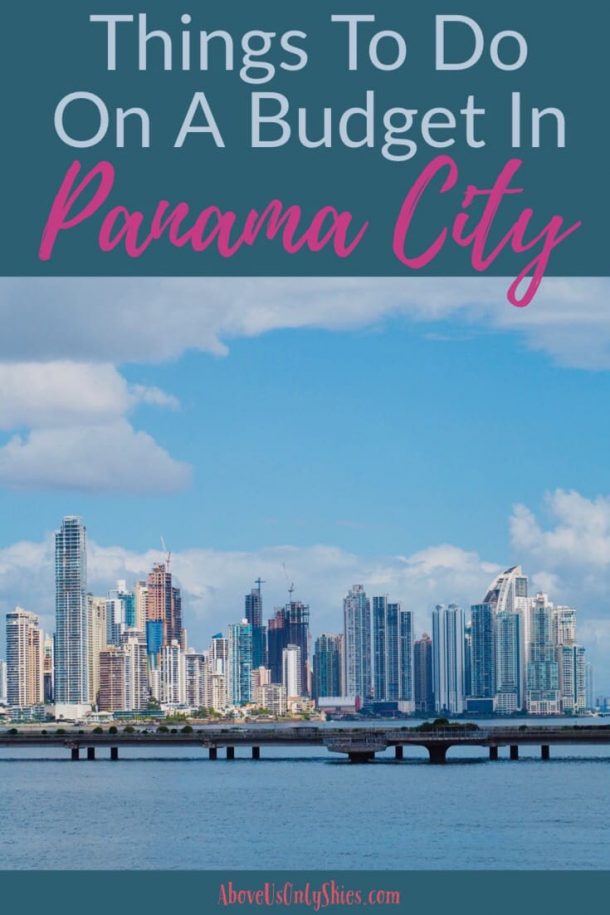The image appears to be the cover of a brochure or book titled "Things to Do on a Budget in Panama City," published by aboveusonlyskies.com. The title at the top is presented in a light bluish-green square with "Things to Do on a Budget" in a lighter color. The phrase "Panama City" stands out in hot pink cursive, slanting to the right, deviating from the standard font. At the bottom of the cover, "aboveusonlyskies.com" is repeated in a stylized, lighter pink font.

The background features a vibrant scene with clear blue skies and numerous puffy clouds. Below the sky, a modern metropolitan skyline adorned with numerous skyscrapers stretches up to the water's edge, which could be a bay or sea. Centrally, a significant bridge spans from right to left, supported by several pylons, suggesting it is a major thoroughfare likely accommodating vehicular traffic. The overall atmosphere of the setting is calm, with no signs of stormy weather.